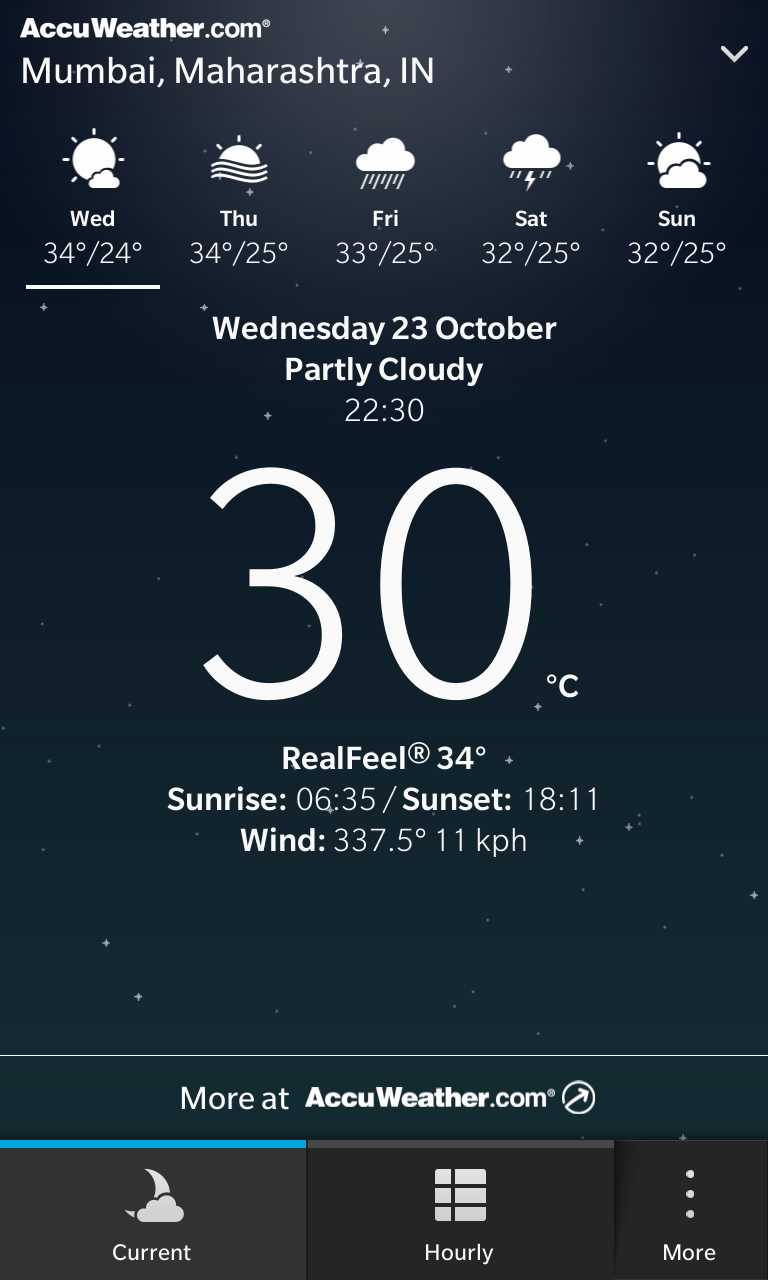This image is a screenshot from the AccuWeather website, specifically providing weather details for Mumbai, Maharashtra, IN. In the upper left-hand corner of the screenshot, the AccuWeather logo and website address, accuweather.com, are prominently displayed. The forecast spans from Wednesday to Sunday, listing both the high and low temperatures for each day.

Centered in the image are the details for Wednesday, 23 October, noting that the weather is partly cloudy. The time is recorded as 22:30. The temperature reads 30 degrees Celsius but feels like 34 degrees Celsius. Below this, it mentions that the sunrise occurred at 06:35 and the sunset took place at 18:11. The wind direction and speed are also provided, indicated as 337.5 degrees at 11 kilometers per hour.

At the bottom of the image, the phrase "more at accuweather.com" is visible, suggesting additional information is available on the website. Three buttons are seen towards the bottom of the screenshot: the "current" button on the far left, the "hourly" button next to it, and a button with three vertical dots labeled "more" on the bottom right corner.